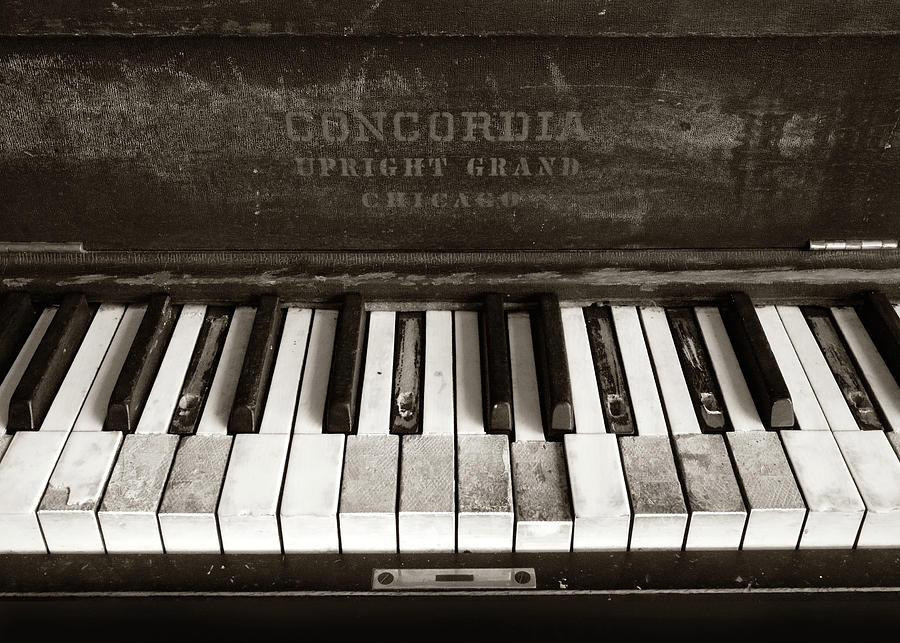This rectangular, black and white photo captures a close-up of an aged Concordia Upright Grand piano from Chicago. The more detailed focal point is the middle section of the keyboard, which is visibly distressed and damaged. The dark brown exterior of the piano, marred with gray markings and dirt, gives a sense of its age and neglect. The white and black keys are in varying states of disarray and decay; many black keys are missing, while the white keys show black stains and broken pieces, some exposing darker interior parts, possibly remnants of glue. The text across the front of the piano, "Concordia Upright Grand Chicago," is in gray and appears faded and worn, further attesting to the piano's long history and disuse.